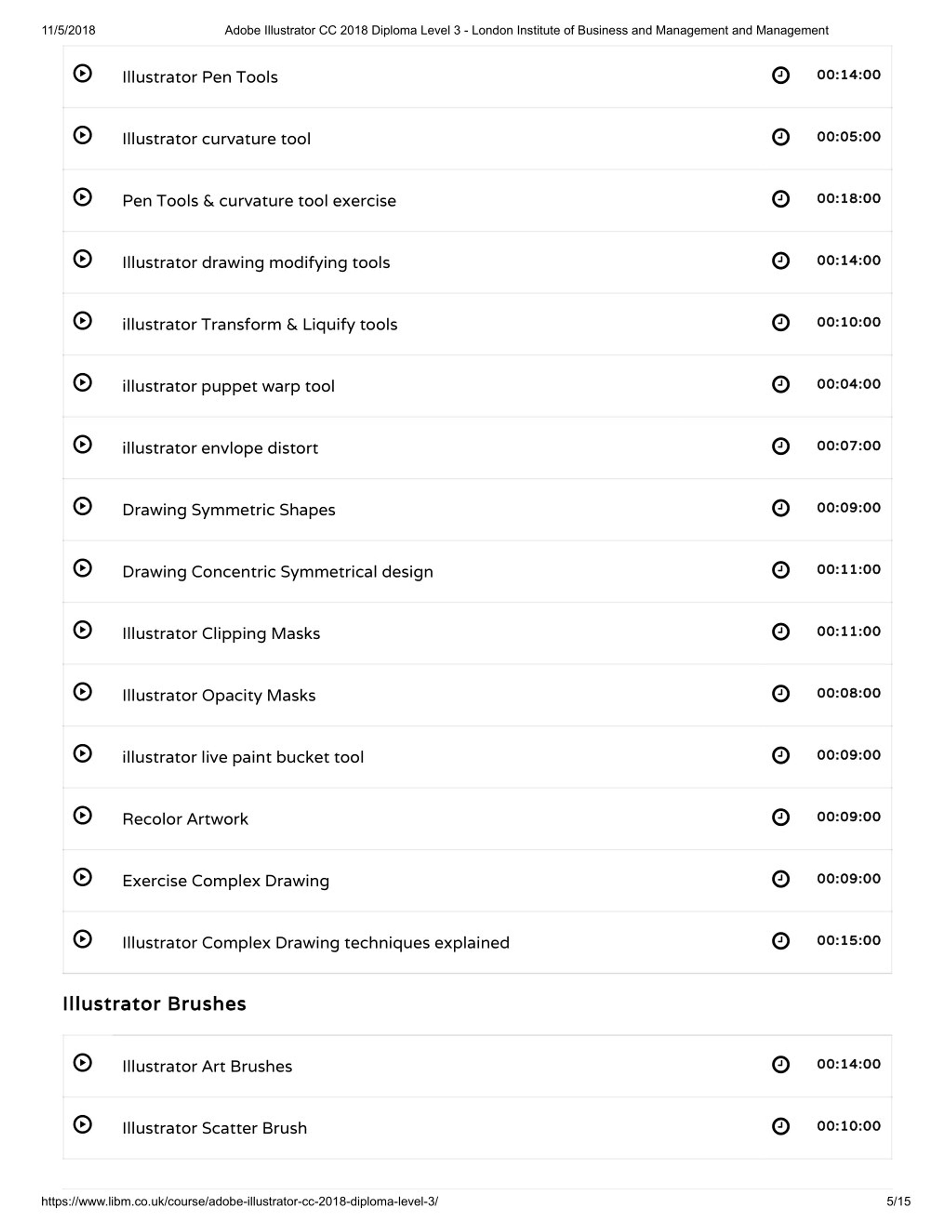The image features a predominantly white background with text detailing a course module for Adobe Illustrator CC 2018, specifically Level 3 of a Diploma offered by the Institute of Business and Management.

In the top right corner, the text reads "Adobe Illustrator CC 2018 Diploma Level 3" and below it, the name of the institute is mentioned. The top left corner displays the date "11-05-2018."

The image lists a series of video tutorials by their titles and durations. The sequence begins with:

1. Illustrator Pen Tools – 14 minutes
2. Illustrator Curvature Tool – 5 minutes
3. Pen Tools and Curvature Tool Exercise – 18 minutes
4. Illustrator Drawing Modifying Tools – 14 minutes
5. Illustrator Transform and Liquify Tools – 10 minutes
6. Illustrator Puppet Warp Tool – 4 minutes
7. Illustrator Envelope Distort – 7 minutes
8. Drawing Symmetric Shapes – 9 minutes
9. Drawing Concentric Symmetric Design – 11 minutes
10. Illustrator Clipping Mask – 11 minutes
11. Illustrator Opacity Mask – 8 minutes
12. Illustrator Live Paint Bucket Tool – 9 minutes
13. Recolor Artwork – 9 minutes
14. Exercise Complex Drawing – 9 minutes
15. Illustrator Complex Drawing Technique Explained – 15 minutes
16. Learn Days
17. Illustrator Brushes – unspecified time
18. Illustrator Art Brushes – 14 minutes
19. Illustrator Scatter Brush – 10 minutes

At the bottom of the image is a URL, "www.libm.co.uk," which redirects to the Adobe Illustrator courses. The bottom right corner indicates the page number, "5 of 15."